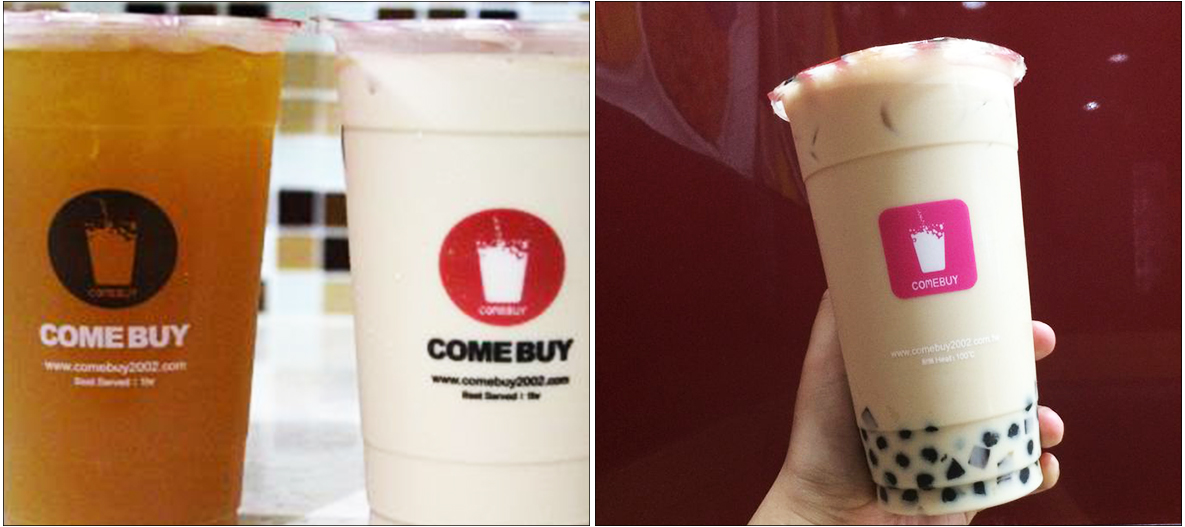This composite image features two distinct pictures showcasing three beverages from the franchise "Comebuy." The picture on the left displays two clear cups placed on a white table against a mosaic tile backdrop. The cup on the left contains an orange liquid with a black logo resembling a cup cutout, surrounded by the words "Comebuy" in white, accompanied by the website "www.comeby2002.com" and additional text underneath. The cup on the right holds a white or tan liquid, featuring a red logo with the same black "Comebuy" inscription and website. The accompanying picture on the right shows a third beverage, a clear cup with a brown coffee-like liquid, held by a left hand in front of a dark red wall. This cup sports a pink square logo and contains black boba pearls at the bottom. Both images emphasize the consistent branding and trademarks of the "Comebuy" franchise across different drink varieties.